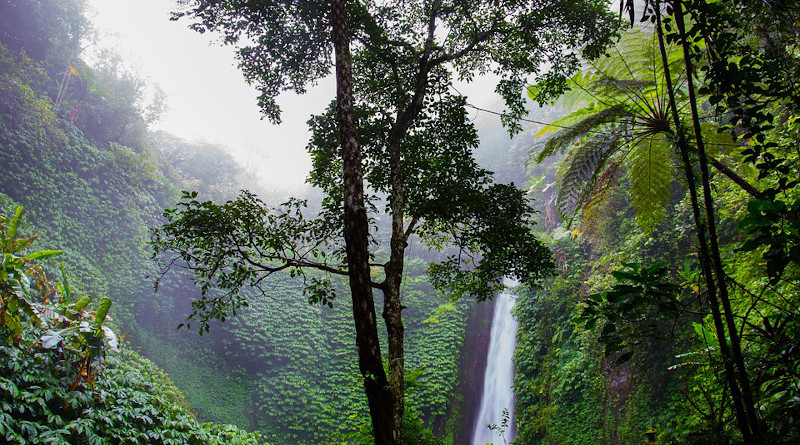The photograph depicts an incredibly vivid and sharp scene of a tropical rainforest, likely resembling the lush greenery of the Amazon. Dominating the composition is a thin, tall waterfall cascading from a rocky, mountainous area slightly off-center to the right. The water appears brilliantly white as it splashes down, though the basin where it lands is not visible. The scene is enveloped in thick, vibrant foliage, with diverse tropical trees and vines blanketing the surrounding cliffs and hills. The center features a prominent tree with abundant leaves at its top, while to the right, there’s a thin tree adorned with what appear to be nuts. Some of the trees show brownish trunks and some white markings. The left side of the image reveals a hazy, foggy sky, possibly cloud cover, breaking through the dense canopy, adding a mystical feel to the entire setting. The entire forest is brilliantly green, illuminated by light filtering through the mist, enhancing the wild and untamed beauty of the rainforest.